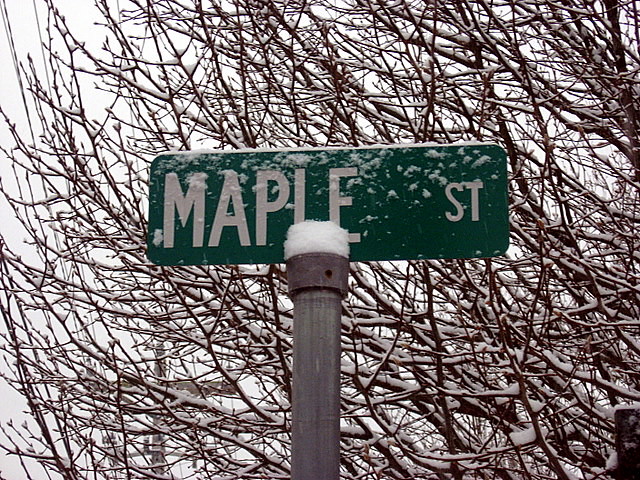In this photograph, the focal point is a green street sign marked "Maple Street" in bold white letters. The sign is mounted atop a metallic gray pole. Snow has delicately accumulated on the upper edge of the pole and is scattered across the face of the sign. Despite the snow, the text remains clearly readable. Surrounding the sign, the barren branches of a tree are visible, each twig encased in a layer of snow. The sky forms a cloudy, overcast backdrop, suggesting a cold day devoid of direct sunlight.